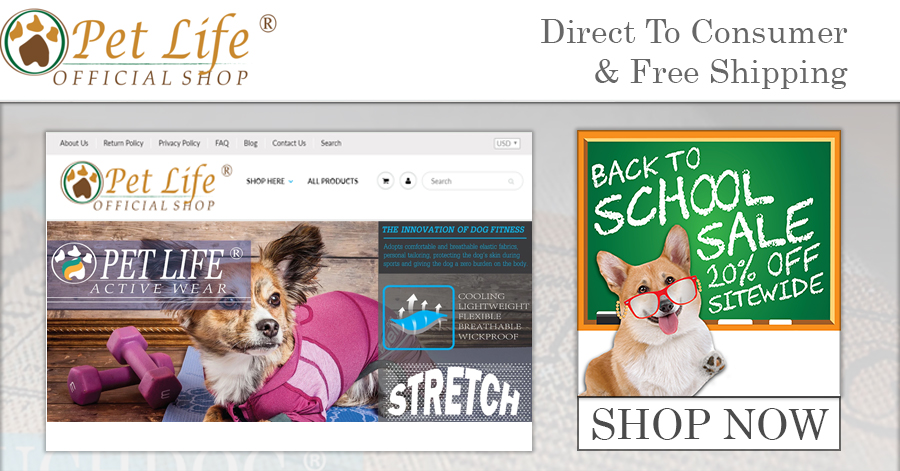### Caption:

Screenshot of the "Pet Life" official website, showcasing various features and promotional elements. The website's title "Pet Life®" is prominently displayed at the top in a mix of brown and orange fonts, with an orange paw print logo encircled in brown and green nearby. Directly beneath these, the words "official shop" are visible. Adjacent to this section, gray text reads, "Direct to consumer and free shipping."

The main content of the screenshot is divided into two sections within gray boxes against a tan background. The first section displays a detailed view of the Pet Life official shop's homepage. This includes familiar elements such as the paw logo, and various submenus like "About Us," "Return Policy," "Privacy Policy," "FAQ," "Blog," "Contact Us," and a "Search" option. Next to the logo, the banner invites users to "Shop Here - All Products" and features a shopping cart icon, another black icon in a white circle, and a white search box.

Below this, there's an image of a small, caramel, white, and black dog wearing a pink onesie labeled "Pet Life Active Wear" in a little purple box. Another blue box highlights "The Innovation of Dog Fitness," followed by descriptive text in blue, mentioning features such as "Cooling, Lightweight, Flexible, Breathable, Wick-Proof, Stretch," with a corresponding image of a blue and gray object with arrows.

The second section features a small blonde and white dog wearing red glasses with its tongue playfully hanging out. It is set against a chalkboard backdrop with the text "Back to School Sale 10% off Sitewide" written in white chalk-like font. At the bottom of this image, a call-to-action button labeled "Shop Now" is displayed.